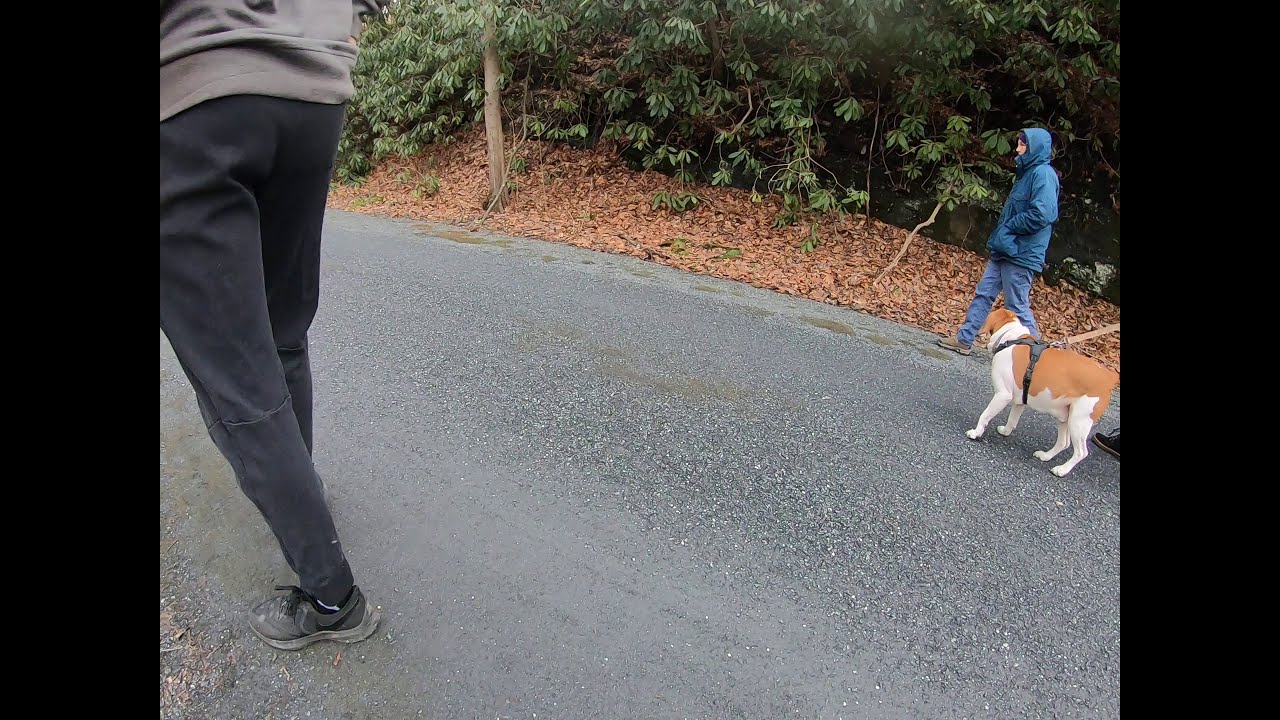In the image, there is a light brown asphalt road that traverses through the countryside, with various patches of vegetation growing through it. The road is lined with dead and dried leaves, along with various trees and green vegetation. Walking on this road are two to three people, with their details partially visible. 

On the left side, the bottom half of a person is seen, dressed in a gray sweatshirt, black pants, and black and gray shoes. Their waist, legs, and feet are visible, emphasizing their movement away from the camera. On the right side, a heavily bundled individual in a blue windbreaker with the hood up, blue jeans, and tan and white shoes, strides along the road. In front of this person is a white and brown beagle wearing a black harness attached to a brown leash. The dog's posture and direction suggest it is looking towards the person in the blue windbreaker. 

The person holding the leash is only partially visible, identifiable by their black shoe. The photo appears to be slightly framed by black rectangles on either side, adding a sense of depth and focus. The entire scene is a snapshot of a peaceful countryside walk, capturing the subtle interaction between people and their environment on an unassuming asphalt road amidst nature.